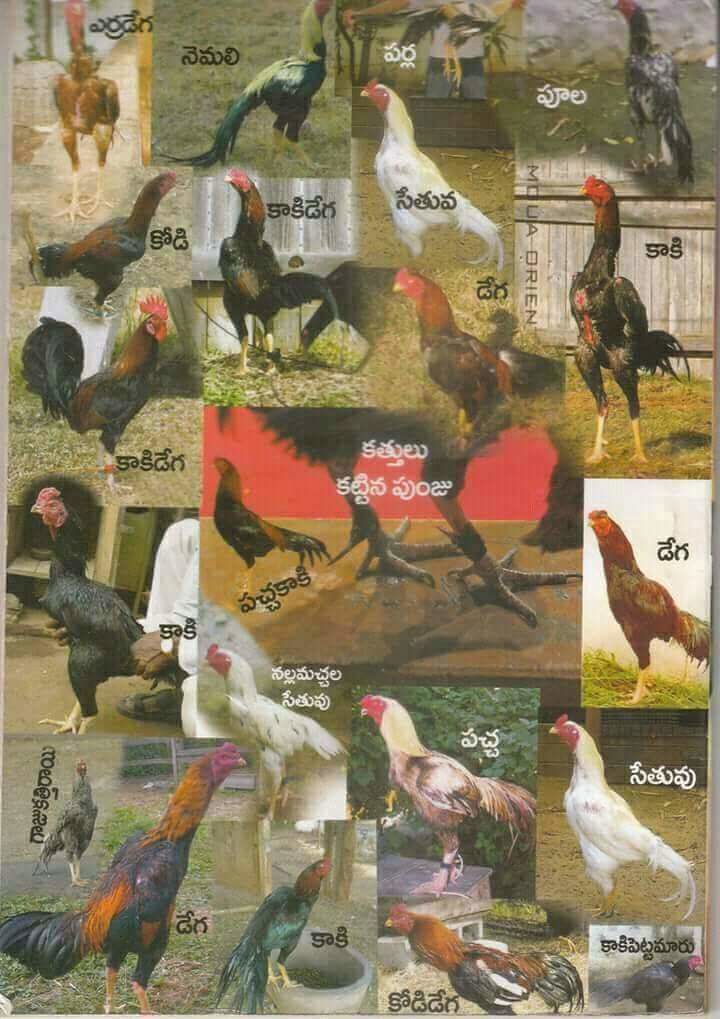The poster is a vibrant collage of various rooster photographs, showcasing multiple breeds and colors. The layout begins with the top row featuring four roosters from left to right, where the third rooster image is notably twice as long as the others. The second row displays two red and black roosters, stacked vertically and slightly smaller than those in the top row. Continuing to the right, another red and black rooster stands upright. Below these, on the left, a man holds a black rooster with its head to the left and tail to the right. Adjacent to this, a large central square image captures the feet of a rooster with a smaller red and black rooster in the background. To the right, a rectangular image showcases a light brown and dark brown rooster. 

The bottom row begins with a small photo of a gray rooster walking towards the camera. Next is an image of the back of a dark brown and black rooster, its head turned to the right. To the right of this, another dark brown and black rooster stands on a pale silver object. The following picture presents a red and black rooster facing left. The row concludes with a final red and black rooster on the bottom right corner, above which a white rooster with its head facing left completes the layout.

Throughout the poster, text in both black and white appears on various images, possibly in a foreign language, against farm backdrops complete with grass and white fences. Some roosters are described to have distinctly colored parts such as black chests, brown necks, and red heads. The poster includes chickens not only of mixed red and black varieties but also white ones with red areas around their mouths, and other combinations like gray and brown. The top right features the words "M-O-U-A D-R-I-E-N" in a transparent brownish font, adding to the poster's diverse array of details.